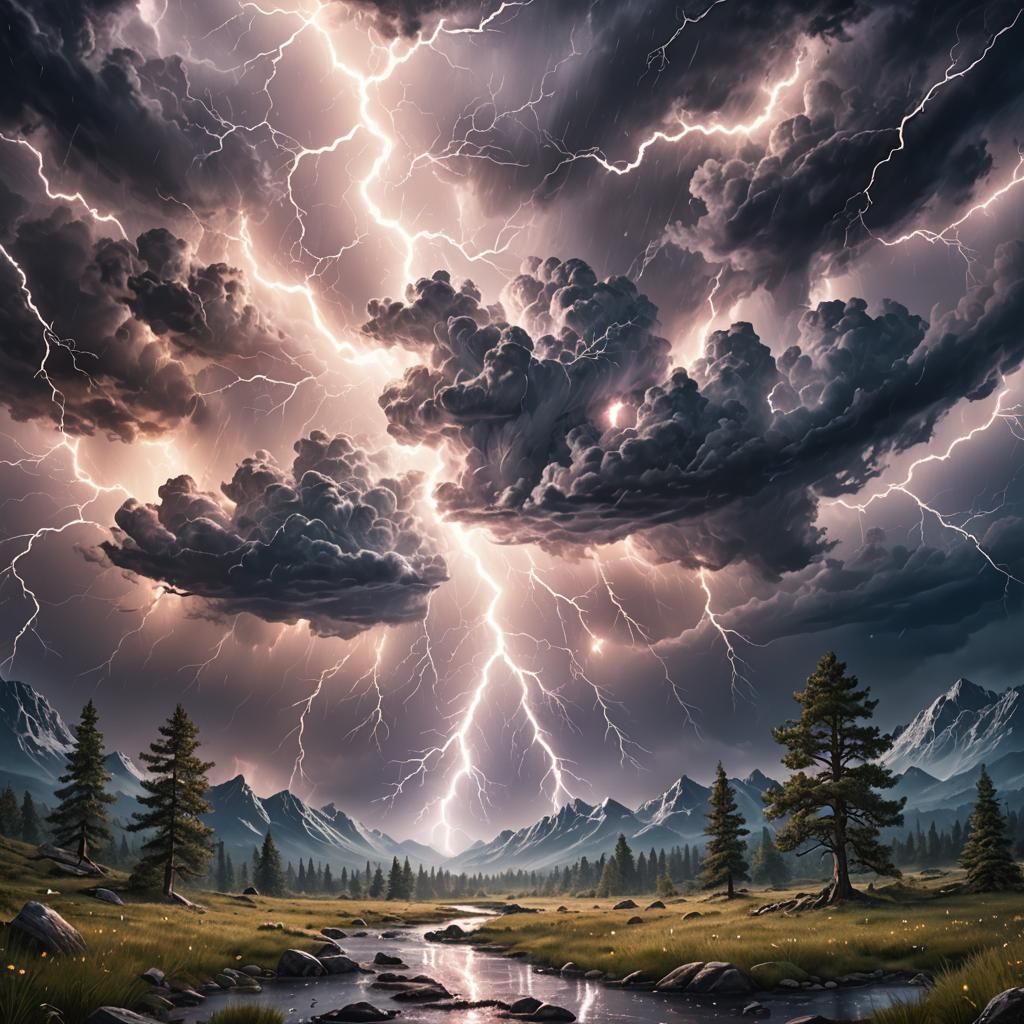In this high-definition image, an intense nighttime storm is captured in an animated style, set in a wooded mountainous region. The top two-thirds of the picture are dominated by a jet-black sky, densely packed with dark black and gray clouds. Purple lightning bolts shoot in every direction, illuminating the thick clouds. Just below this dramatic sky, a mountain range colored in shades of bluish-gray stretches across the horizon. In the foreground, a small creek winds from the bottom of the image toward the skyline, with a slight break at its bottom flowing to the right. Flanking the creek, patches of grass and trees add detail; two trees stand on the left side, while three trees on the right side draw closer. Behind these foreground trees, a continuous row of trees spans the background, completing the scenic yet stormy landscape.